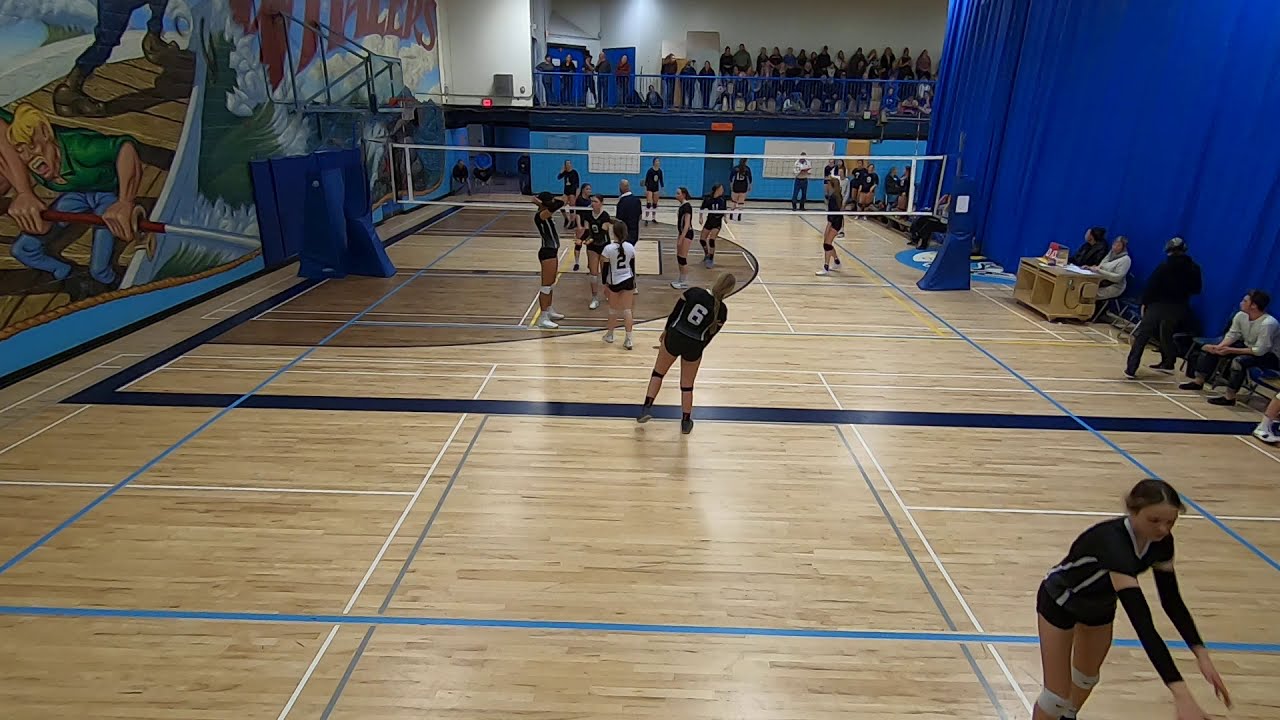The photograph captures an intense high school women's volleyball game taking place indoors in a gymnasium. The scene is set on a wooden basketball court, divided by a white volleyball net. Players from both teams are geared up in black jerseys and shorts, with some sporting knee braces, actively engaging in the game. In the foreground, one player reaches out, poised for action. 

Spectators fill a raised walkway in the background, peering down to catch the on-court excitement. The gym is vividly decorated: the left wall features an ornate mural depicting a muscular man rowing a boat, while on the right, a large blue curtain divides the court. Referees and judges are strategically positioned in front of the curtain, overseeing the match. The rich details in the image highlight the energy and enthusiasm surrounding this high school sporting event.